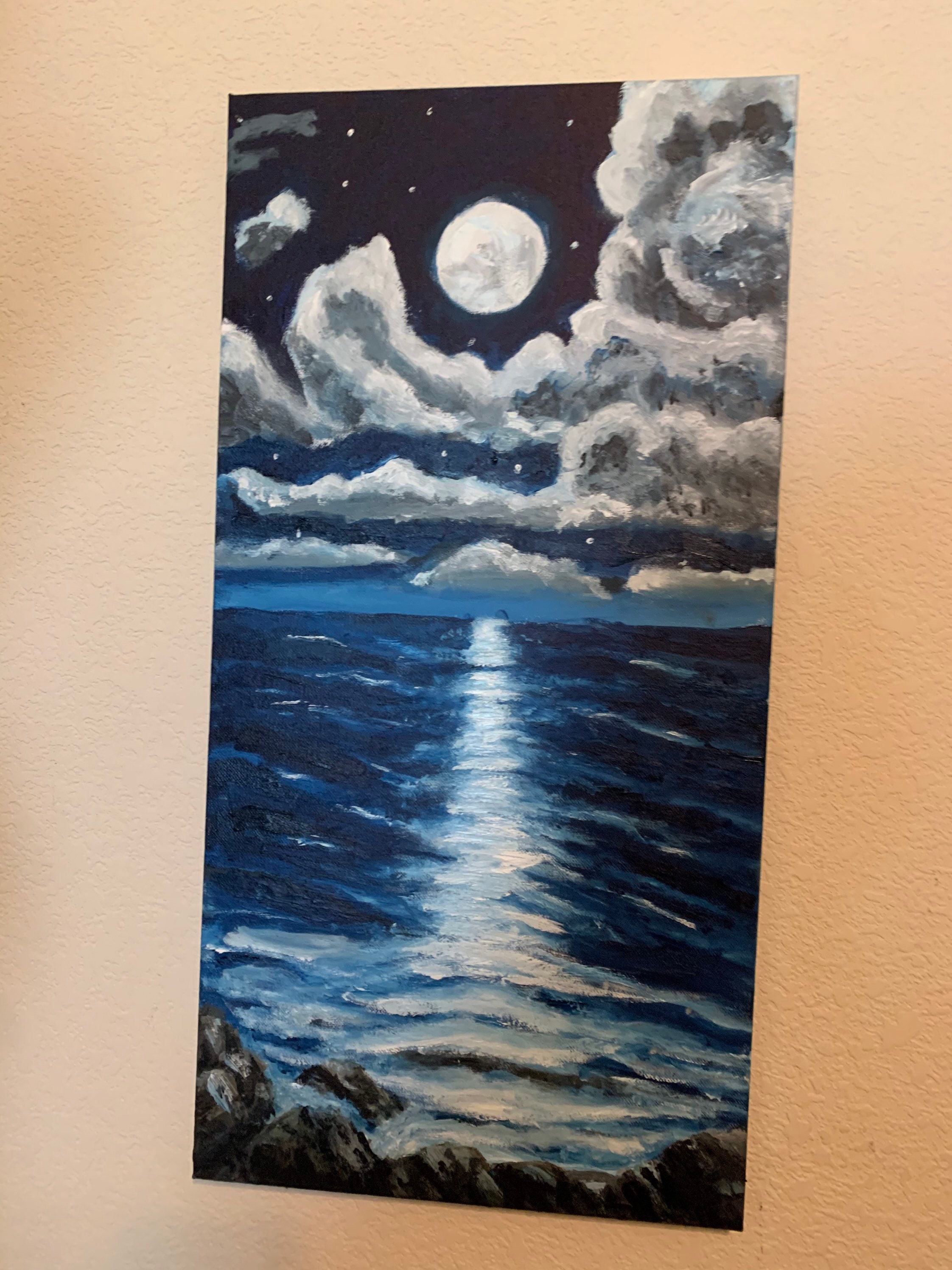This image depicts a photograph of a painting displayed on an orange-ish to rose-colored background wall, slightly tilted at a diagonal. The painting itself is a vertical rectangle, capturing a serene nighttime seascape in shades of blue and white. At the top half of the painting, a dark night sky is partially obscured by fluffy, gray clouds, leaving open patches that reveal a scattering of stars. The moon, prominently featured in the upper center, casts a luminous reflection on the ocean, creating a glowing, expanding path of light on the deep blue waves that leads towards a rocky shore visible at the bottom of the painting. The moonlight's interplay with the waves, cresting with white foam, creates a sense of movement and tranquility, inviting viewers to feel as though they are standing at the water's edge.